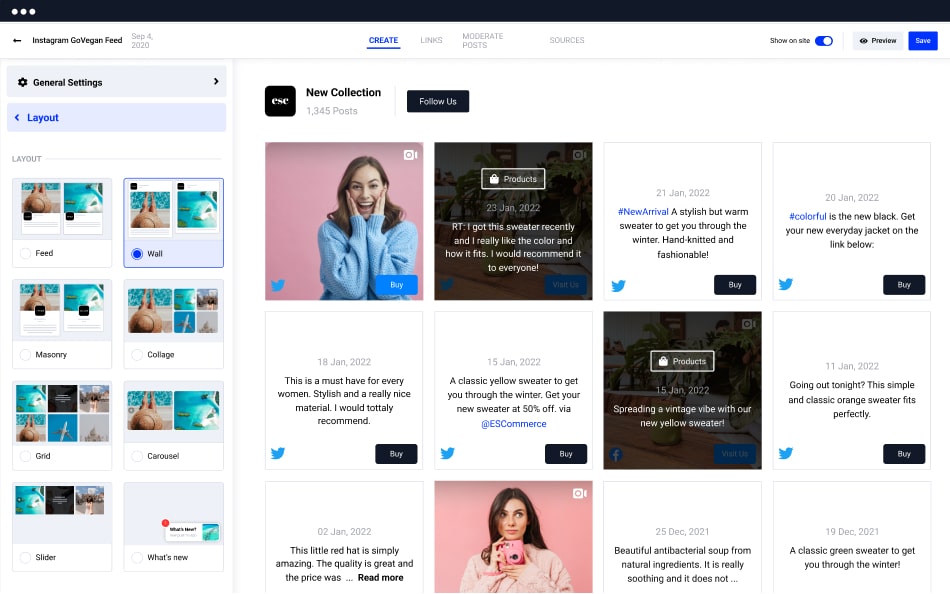The image depicts a complex social media interface, likely from Twitter but incorporating elements resembling Instagram settings. The top section features a long, black bar with a menu button. Immediately underneath, smaller text reads "Instagram settings feed," suggesting a potential integration or link to Instagram.

Below this, the interface presents a series of menu options including "Create," "Sources," "Moderate Post," and an option for marking items as new. These options are contained within a box that appears to be on the left side of the screen.

To the left, there is an array of images displayed in a collage format. The images appear to be the same but shown with different filters. One prominent image in the collage shows what might be a woman, although this is unclear. Adjacent to it is a light blue image, possibly depicting a beautiful body of water, though it is very small and not particularly clear. Another section seems to depict beach-related content, possibly featuring an animal or a shell against a background of a brown substance.

Further down this section, there are additional random images, one with a black background and another with an aerial perspective. The top of these sections is labeled "General settings and layout," with options related to filters and positioning.

On the right side of the screen, another collection of images is displayed under the heading "New Collection." The first row prominently features a young woman with long brown hair, wearing a blue sweater and smiling brightly with her hands on her cheeks. 

Below this, additional rows contain images with white backgrounds and black captions, though the text is too small to be legible. The final row mirrors this format but includes an image of a different woman with long dark hair and a neutral expression. She is wearing a pink shirt and holding a pink camera.

Overall, the image appears to blend elements from multiple social media platforms, highlighting various content and user interface options.